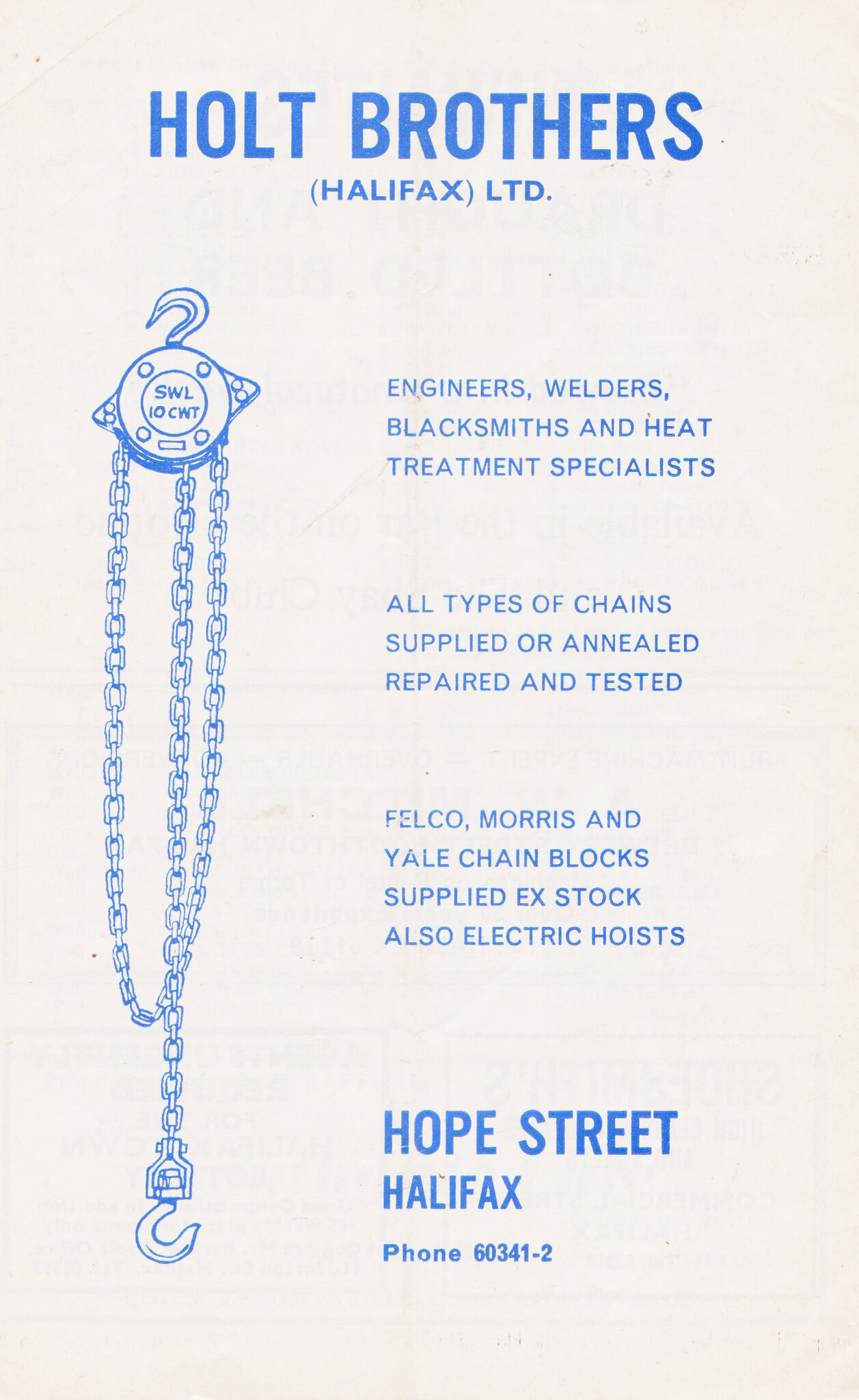The image is a full-page advertisement with a creamy white background and blue ink for both text and illustrations. At the top, it reads "Holt Brothers Halifax Ltd." Below that, in smaller text, it describes their services: "Engineers, Welders, Blacksmiths, and Heat Treatment Specialists." The ad continues with the message, "All types of chains supplied or annealed, repaired, and tested. Felco, Morris, and Yale chain blocks supplied ex-stock. Also electric hoists." Towards the bottom, it lists the address as "Hope Street, Halifax" in bold blue text, followed by the phone number "60341-2." On the left side of the page, there's a detailed illustration showing a chain wrapped around a pulley, with a hook hanging from the bottom end of the chain.